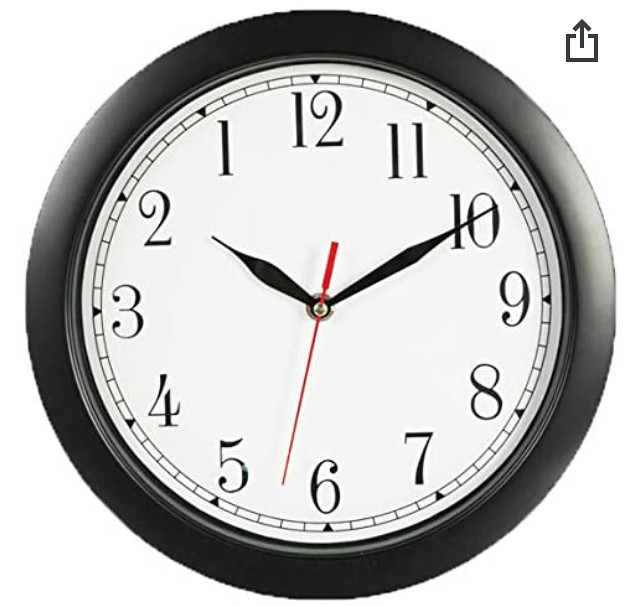This image features a prominently displayed white-faced wall clock that occupies the majority of the frame. The clock is encircled by a black outer border that runs along its circumference. Notably, the clock face displays a full set of numbers from 1 through 12 arranged in a counterclockwise fashion, creating a unique reversed appearance. For instance, the number 1 is positioned where 11 usually is, the number 2 where 10 would typically be, and so on, culminating with 12 at the top and 6 at the bottom.

The clock has three hands: a short black hour hand, a longer black minute hand, and a distinct red second hand. The black hour hand is just past the 2, indicating it’s a little after 2 o'clock. The black minute hand points towards the 10, suggesting approximately 50 minutes past the hour. The red second hand is positioned between the 5 and the 6, denoting the precise counting of seconds. Additionally, an interior black double-wide, parallel strip runs around the inner circumference of the clock, adding to its detailed design.